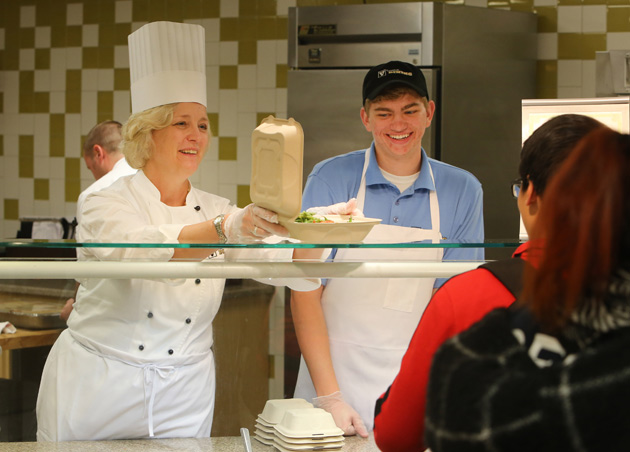The image depicts a bustling scene inside a cafeteria or college dining hall. At the heart of the image is a woman donning a tall white chef's hat, a white chef's coat, and a white apron tied around her waist. She wears clear plastic gloves and is presenting an open, khaki-colored takeout box, seemingly filled with greens, possibly a salad, to a customer. The customer, a woman with red hair in a ponytail, wearing glasses, a red shirt, and a backpack, is positioned in the lower right-hand corner of the image, facing away from us.

Next to the chef, there stands a young man with a light blue polo shirt, a full-length white apron, and a black hat, his short light brown hair peeking out from underneath. He is looking at the food being presented with a smile on his face. The setting features a glass counter with a glass shelf above, through which the food is being handed to the customer. The overall ambiance suggests a friendly and professional environment, emphasizing the cafeteria's commitment to hygiene and customer service.